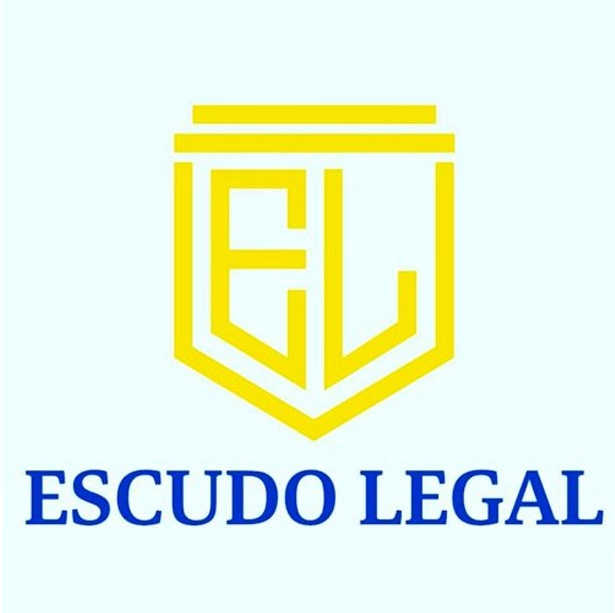This is a vertically rectangular image with a smooth, very pale blue background. At the center of the image is a large, bright yellow logo. The logo has an intricate design, resembling a modified cube or a baseball diamond shape. It features two horizontal lines at the top, with the bottom half forming an inverted triangle-like shape. Embedded within this geometric structure are the initials "E" and "L," which are creatively integrated to complete the overall design. Beneath the logo, in large dark blue text, are the words "Escudo Legal." The text and initials in the logo align to signify the name, enhancing the cohesive branding of the image.